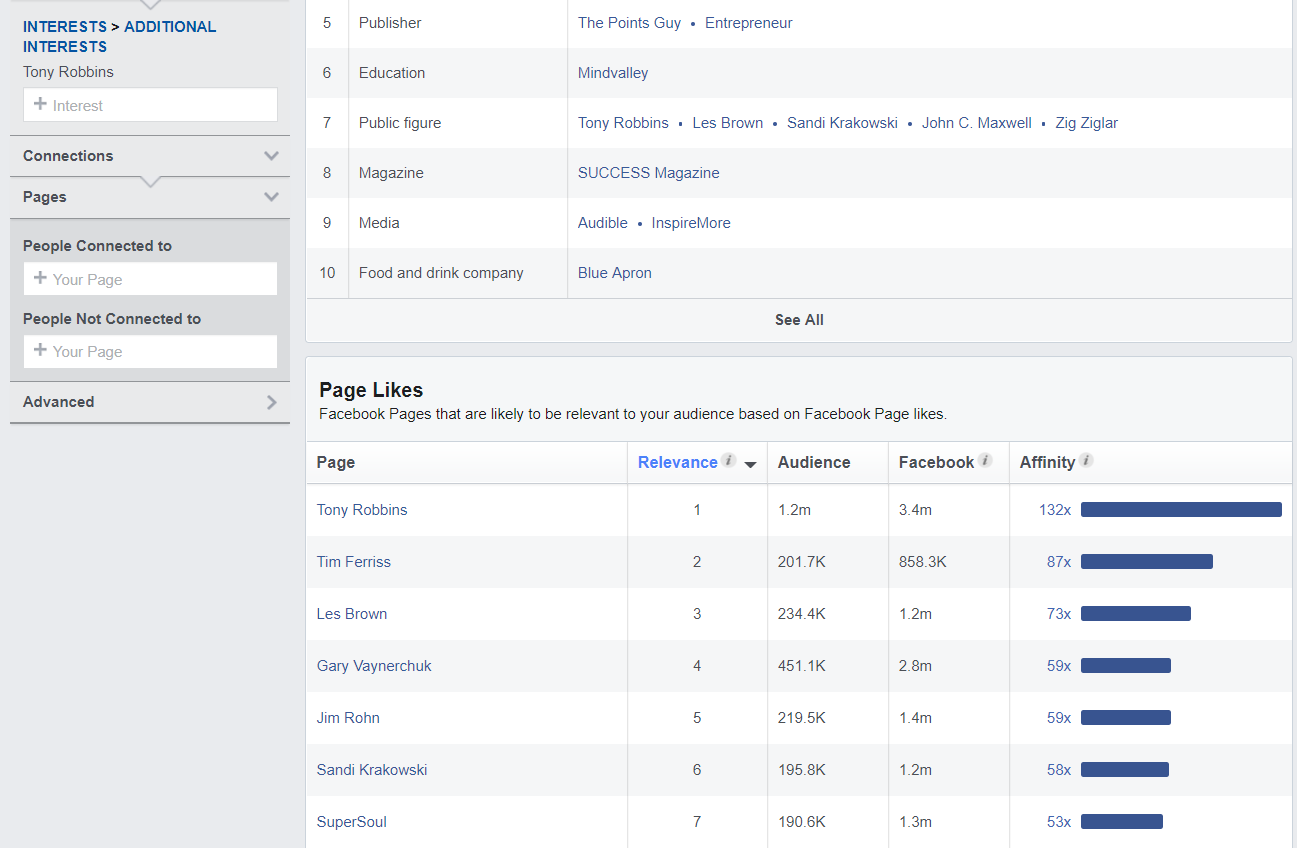The image is a detailed screenshot of an informational page that appears to be analyzing interests and relevant connections for an audience. At the top left corner, it prominently mentions "Interest" and "Additional Interest," with "Tony Robbins" listed above them. In the middle section, the first entry starts with "Publisher," indicating interests such as The Points Guy, Entrepreneur, and Mindvalley. It also lists public figures like Tony Robbins, Les Brown, Cindy Krakowski, John C. Maxwell, and Zig Ziglar, alongside outlets like Success Magazine and Audible. Additionally, categories such as "Education," "Media," "Inspire More," and "Food and Drink Company" with Blue Apron are noted.

Moving further down, the "Page Links" section suggests Facebook pages relevant to the audience's interests, based on their page likes. The highlighted pages include Tony Robbins with a relevance score of 1, an audience of 1.2 million, and an affinity score of 132x. Another notable entry is Tim Ferriss, ranked 2, with an audience of 201.7k.